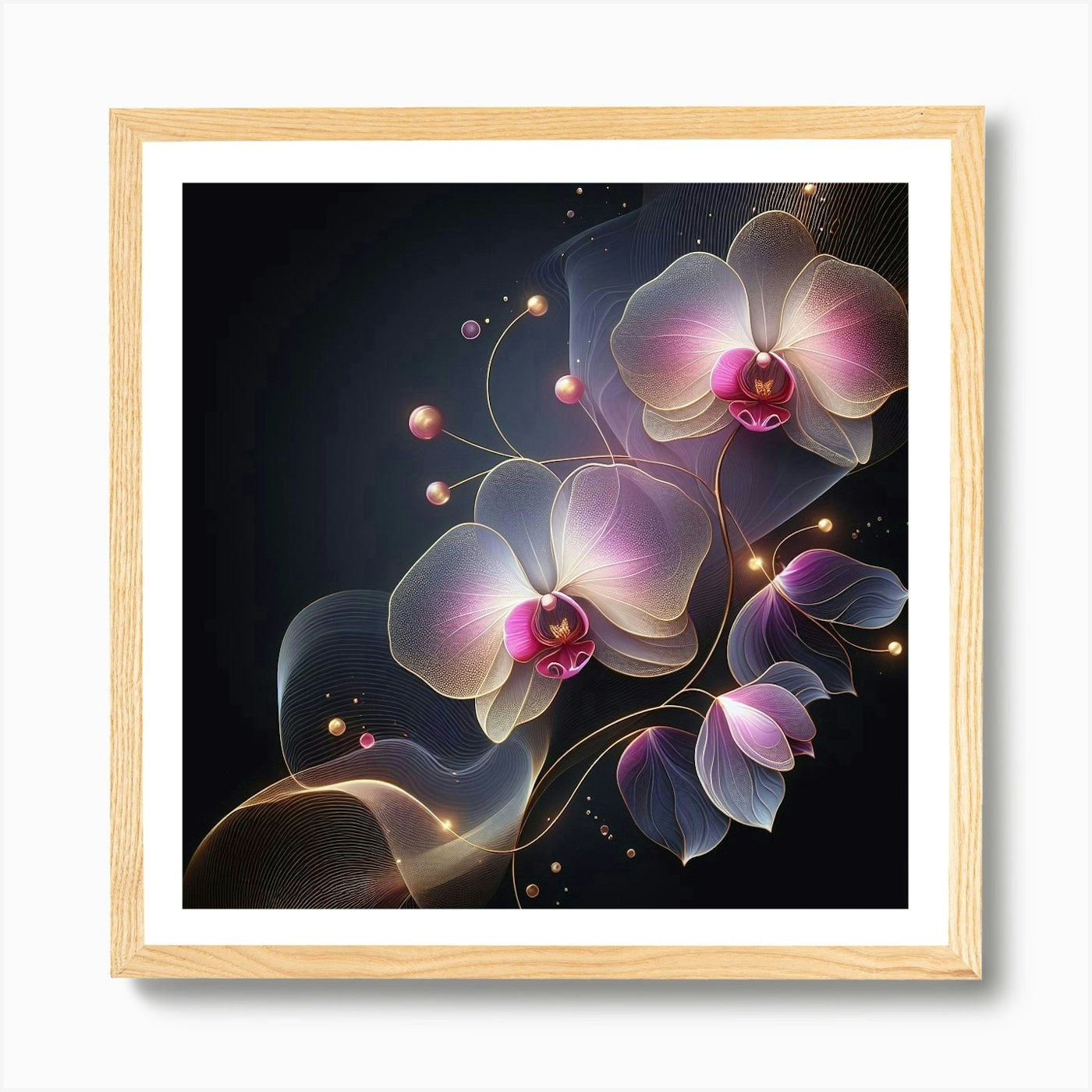This image depicts a computer-generated artwork presented in a square, light natural wood frame. The frame features a thin white inner border and appears to be placed against a solid white background, accented by a digitally added shadow on the right and bottom sides, enhancing the 3D effect. The central artwork showcases a digital drawing of multiple flowers with intricate details. The flowers have pinkish-purple centers with white petals imbued with light pink hues, resembling orchids. These blooms are attached to gold stems, some of which bear pearlescent-like balls and smaller golden balls. The black background of the drawing further highlights the flowers and the golden decorative elements, including scattered golden dots. The overall composition, from the frame to the flowers and their ornamental details, clearly indicates the use of digital editing and design techniques.